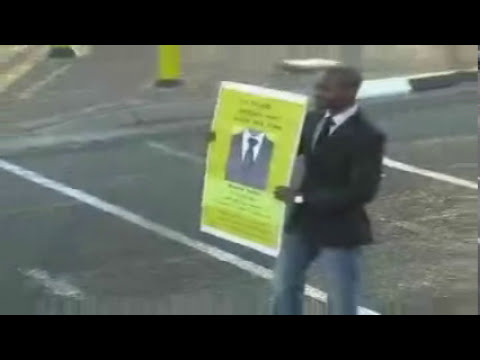The blurred image features an African-American man standing slightly to the right of center, wearing a black suit coat, a black tie, a white collared dress shirt, and blue jeans. He also has a black watch with a silver face on his wrist. He is holding up a poster with both hands, his left hand slightly higher than his right. The poster displays a suit, similar to what he is wearing, consisting of a black sports coat, a black tie, and a white shirt. Text appears above and below the suit image on the poster but is illegible due to the low resolution of the photo. The background is yellow, and the scene appears to be set in a parking lot, as evidenced by the gray pavement and white-lined parking spaces. Additionally, there are horizontal black bars at the top and bottom of the image, reminiscent of letterbox formatting, with a lime green pillar visible in the back left.